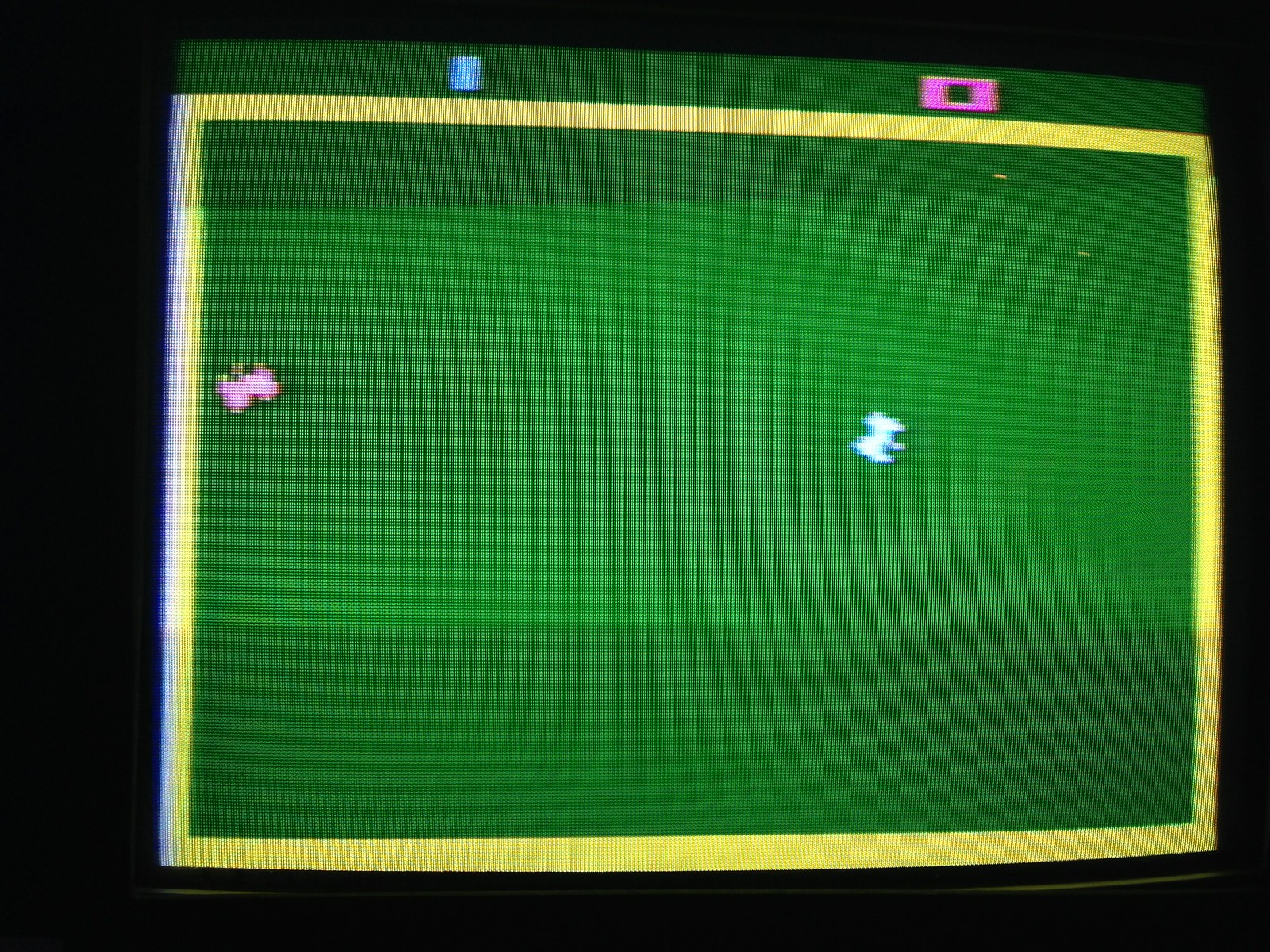The image captures the screen of an older analog tube television, characterized by its prominent back and lower display quality. The content displayed on the TV appears to be an elementary video game, reminiscent of early 1980s computer games or even earlier. The screen's background is dominantly green, with a thin yellow border framing the central area. On the top of the screen, there's a blue, blocky number "1" on the left and a similarly styled pink "0" on the right, suggesting the score of a game. Within this framed area, towards the center left, is a pink irregular blob, and on the center right is a white irregular blob, both hinting at the simplistic graphics common in vintage video games. The black area surrounding the game on the television screen highlights the primitive and basic display, enhanced by visible scan lines indicative of photographing or filming an old screen.